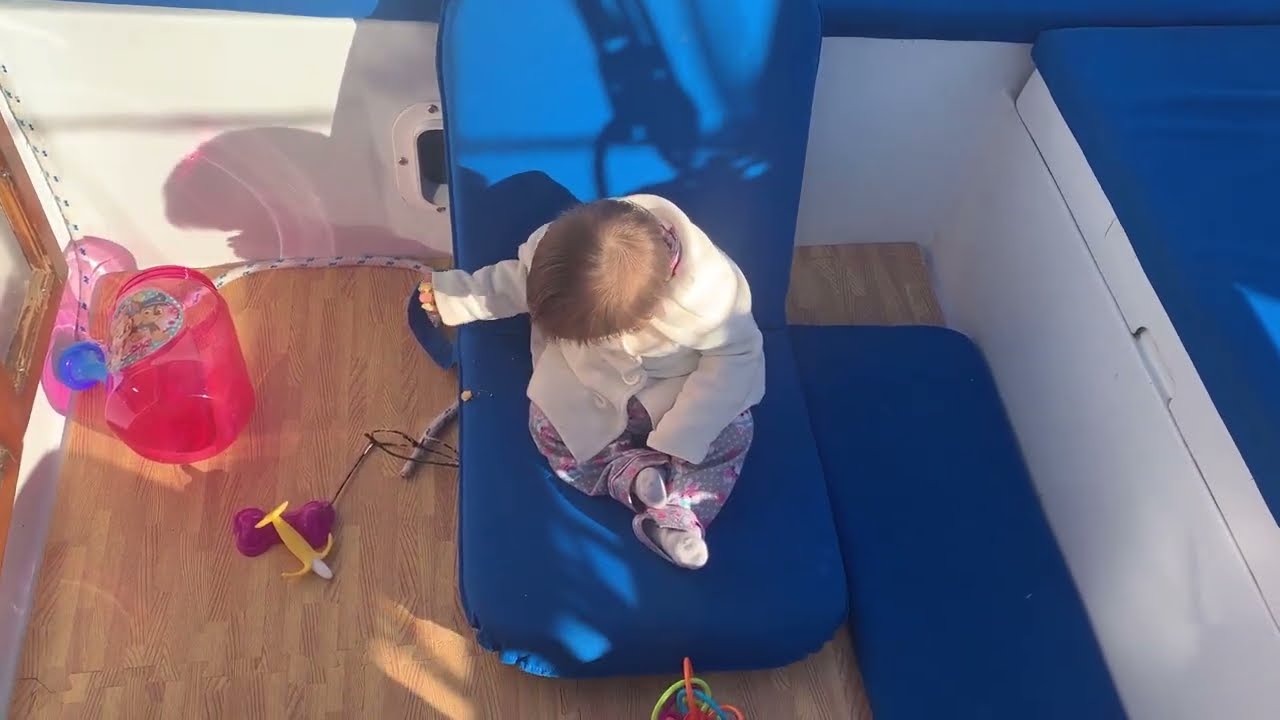The image depicts an overhead view of a toddler girl seated on a blue cushioned chair, situated on what appears to be a boat with black wooden decking. The toddler, with blonde hair and wearing a white long-sleeve shirt or button-down jacket paired with pink and white pants, is looking down towards her left as if she might have dropped something. Surrounding her are various toys, including a partially transparent pink bucket with a character on it to her left and nearby, a yellow toy resembling a banana, a light purple item that could be a ball or bone, and an item that looks like a pair of glasses. The play area is colored with a mix of blue, white, and an assortment of other light hues.